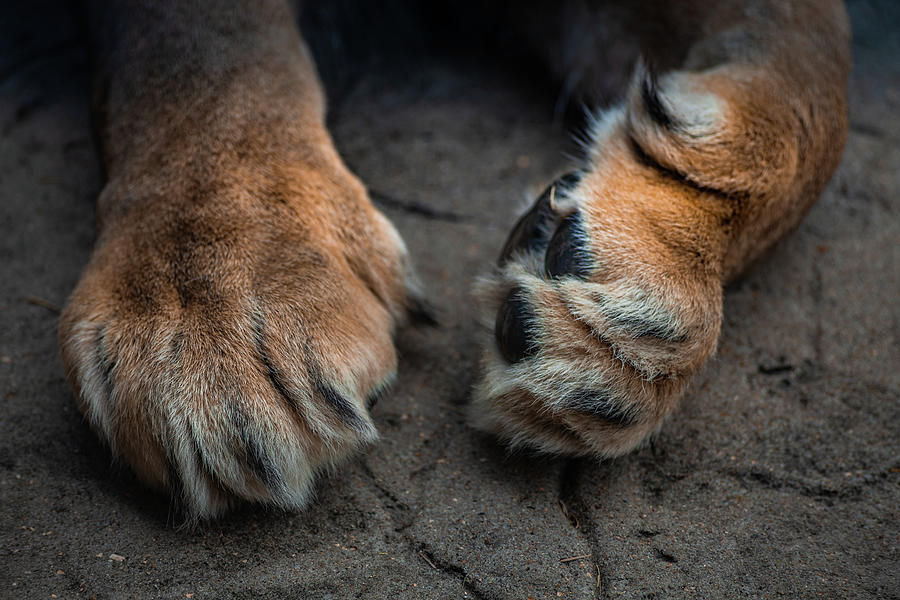The close-up rectangular photograph, approximately five inches wide by three inches high, captures the front paws of a large feline, likely a lion or possibly a tiger, resting on a distinctive ground. The ground itself, visible from top to bottom, is a gray, stone-like surface riddled with tiny divots, lines, sand grains, and filament fragments, lending it a textured, almost man-made appearance reminiscent of a zoo setting.

The feline's paws dominate the image, emerging from the top of the frame. The fur on the paws is a rich orange-brown, with the color lightening to white near the claw areas. The left paw faces downward, with its pad resting on the ground, while the right paw is angled sideways, exposing the thick, dark brown, almost black pads and a hint of a black claw near the dewclaw area. The overall coloration of the fur includes shades of dark brown, light brown, and darker brown spots, blending seamlessly into the sandy, charcoal-hued backdrop. The image focuses solely on the paws and forearms of this majestic creature, highlighting the intricate details of its fur and the rugged texture of the surface below.